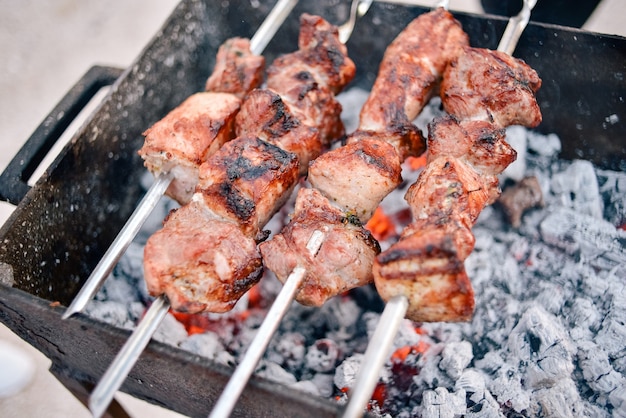This detailed, up-close photograph captures a charcoal grill featuring four metal skewers arranged vertically with a slight slant to the right at the top, each loaded with pieces of meat. The metal skewers, possibly holding chicken or pork, span across a deep black basin grill that appears to be cast iron, showcasing its handle on the left side. The coals within the grill have mostly burned out to a grayish-white ash, though a few glowing red embers remain visible. The skewers display varying numbers of meat pieces, with the far left skewer holding two pieces, the middle left four, the middle right three, and the far right four pieces. The meats are in different stages of cooking, exhibiting black marks and caramelization indicating they are nearing completion. The primary colors of the image include the grayish-brown hues of the meat, the black of the grill, and the gray and orange tones of the embers, combining to create a photorealistic and appetizing scene.